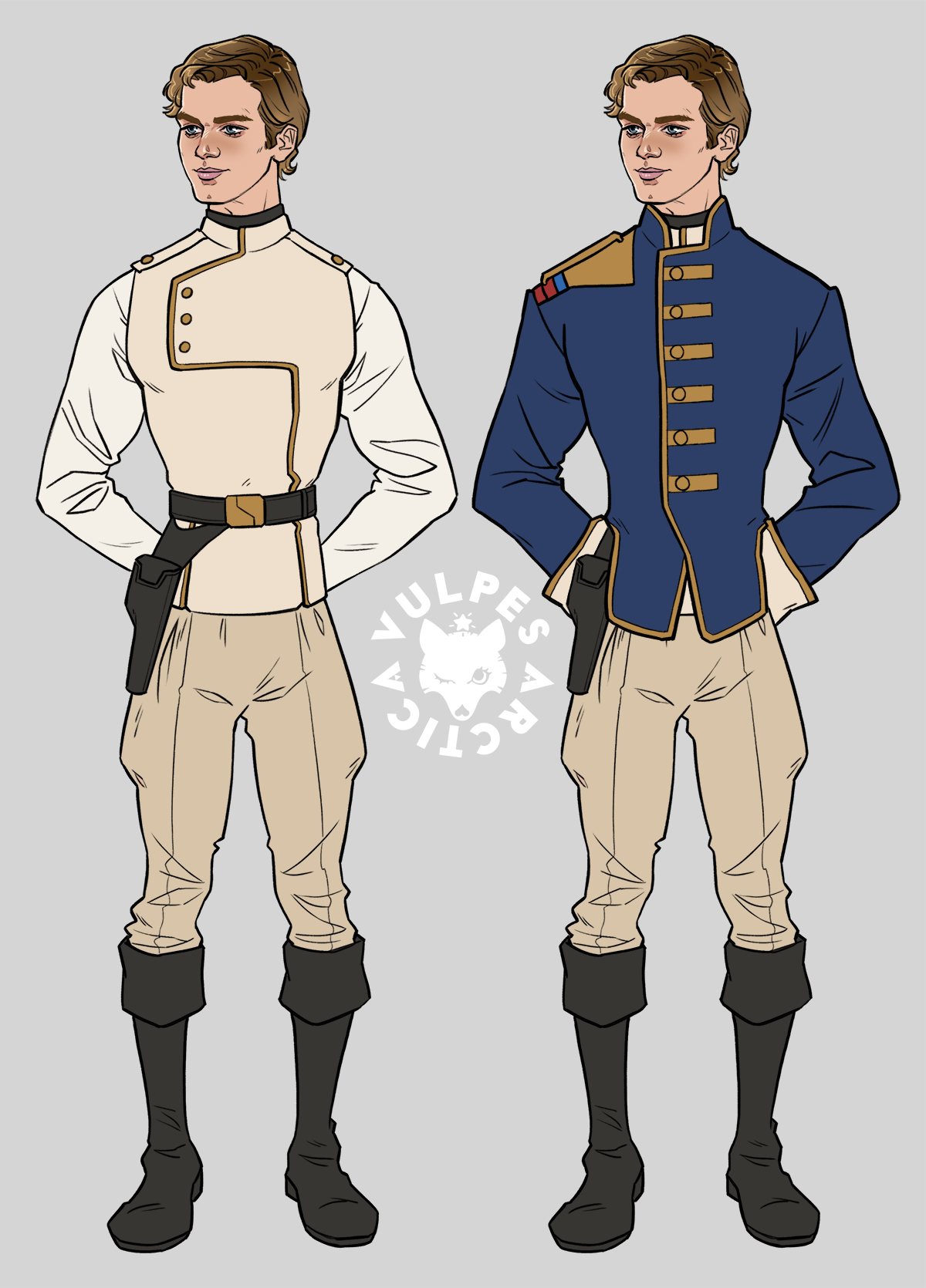The image depicts a digital, animated illustration featuring two nearly identical young men showcasing character development or design. Both characters, positioned against a gray background, have curly brown hair, blue eyes, and clean-shaven faces with a muscular yet slim physique. They stand at attention with their hands behind their backs and both wear beige pants tucked into black, knee-high boots, complemented by a gun holster on their hip.

The significant difference lies in their attire. The character on the left is dressed in a white shirt, over which he wears a beige sleeveless, high-neck jacket with side buttons and a waist belt. In contrast, the character on the right dons a vintage royal blue military-style jacket with golden buttons down the front, badges on the shoulders, and white cuffs with gold trim. A logo featuring a wolf's head with the text "V-UL-P-E-S" and "arctica" appears between the two figures, adding further detail and context to the visual narrative.